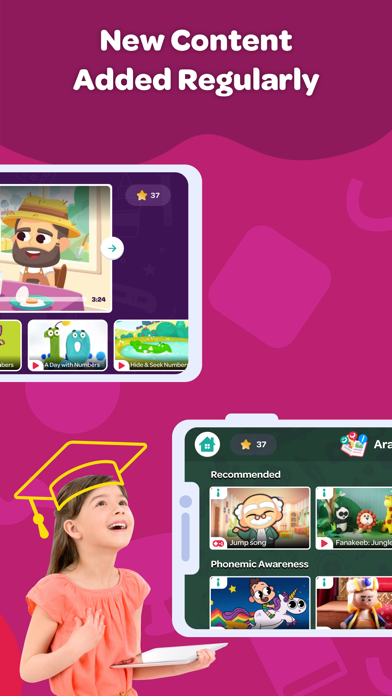The image is a vibrant screenshot of a website, featuring a colorful background with a gradient transitioning from red at the top, through dark pink, to light pink, interspersed with abstract images. Centered at the top, bold white text announces, "New Content Added Regularly."

In the subsequent section, a white tablet is displayed horizontally, showcasing cartoon characters likely from educational material. The screen reveals numerous thumbnails of videos, identified by the presence of red play buttons. One of the highlighted video titles is "A Day with Numbers: Hide and Seek Numbers."

Towards the bottom right-hand corner, another white tablet is depicted on its side, displaying a collection of recommended educational videos focused on "Phonemic Awareness."

At the bottom left-hand corner, there is an image of a little girl with light skin and long brown hair, wearing a coral-colored shirt and possibly a belt. She's illustrated holding a tablet in her left hand and is adorned with an imaginary graduation cap, symbolizing learning and achievement. This imagery reinforces the educational theme, suggesting she is engaged with the tablet's content, particularly in areas of math and reading.